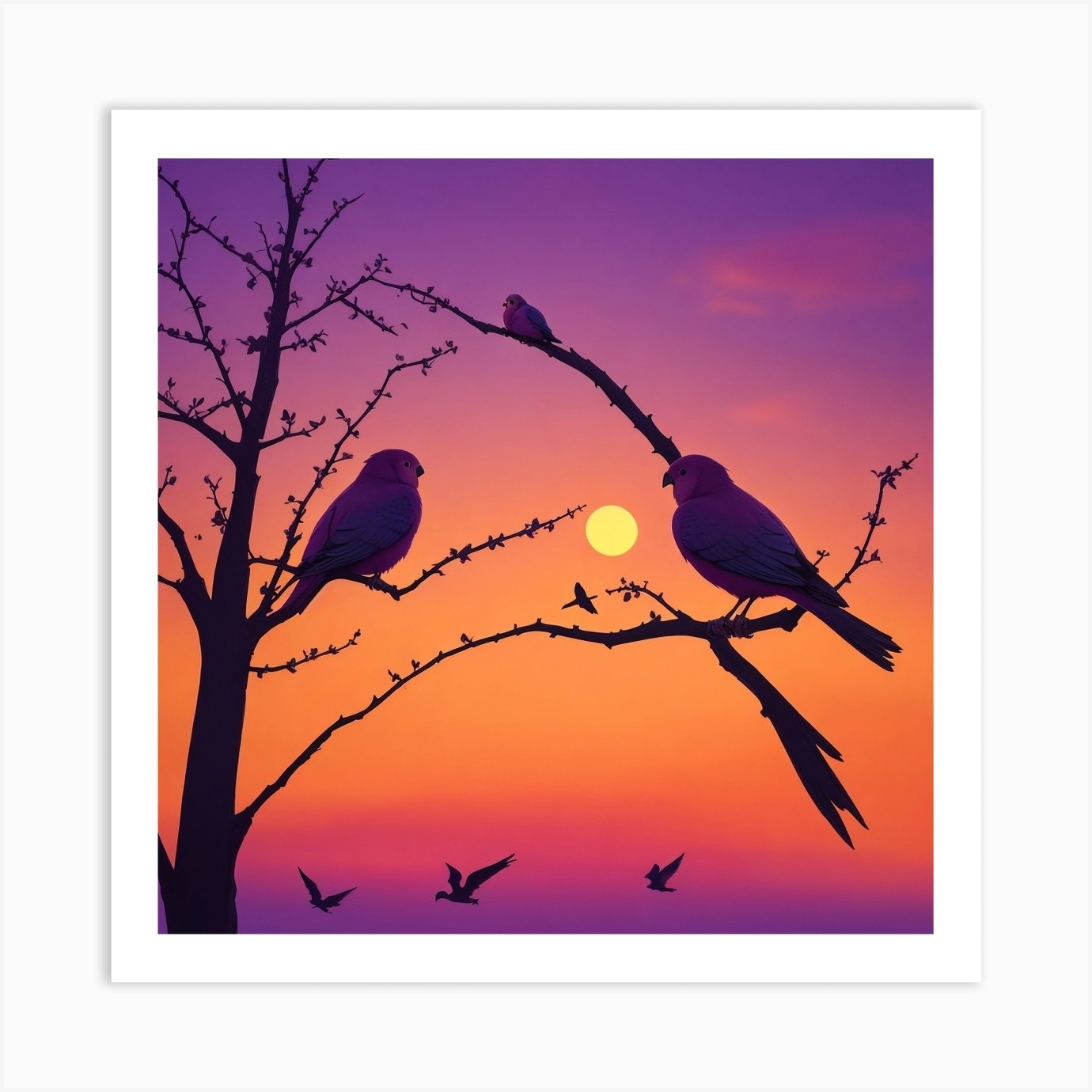This image captures an early springtime scene featuring a tree with budding branches extending from the bottom left and extending to the right, eventually disappearing off the top of the image. The tree's branches split into smaller limbs, with some moving to the left and others to the right. The central focus is a trio of purple-hued birds with gray wings. One bird is perched on a longer branch near the lower part of the tree, facing away slightly to the left, while another bird, also facing away but slightly to the right, is perched closer to the tree's trunk. A third, smaller bird appears further away atop a higher branch in the center-top of the image.

The background presents a gradient sky transitioning from light purple at the top to orange near a round yellow sun positioned to the left of the bird on the lower branch. Below the sun, the gradient shifts through pink hues and back to light purple at the bottom of the image. At the base of the image, three birds are captured in mid-flight, moving from right to left. The image is framed with a white border on the top, left, right, and bottom. The overall scene suggests either a sunrise or sunset, inferred from the warm color palette and the position of the sun. This serene landscape blends the delicate new growth of spring with the tranquil motion of birds, creating a picturesque moment in time.